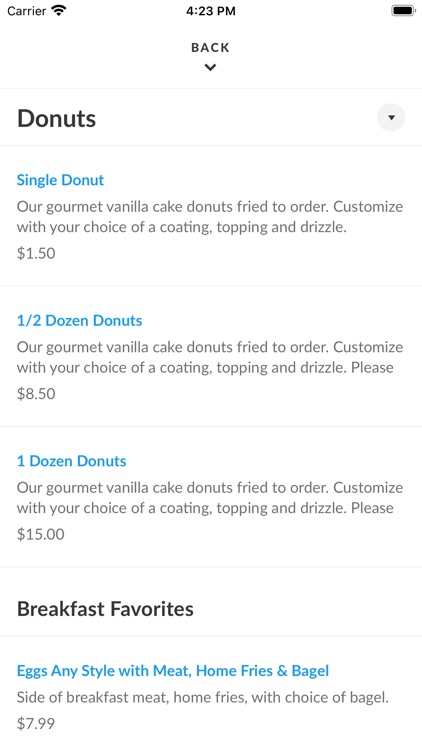Caption:
"The image showcases a variety of gourmet vanilla cake donuts, fried to order and customized with a choice of coatings, toppings, and drizzles. The selection includes options for purchasing a single donut ($1.50), half a dozen donuts ($8.50), or a full dozen donuts ($15). Additionally, the image features a breakfast menu with favorites such as eggs cooked to any style, accompanied by home fries and a bagel, priced at $7.99. The backdrop captures a busy scene, likely indicative of a popular bakery or café, where patrons enjoy a range of freshly made treats and breakfast items."